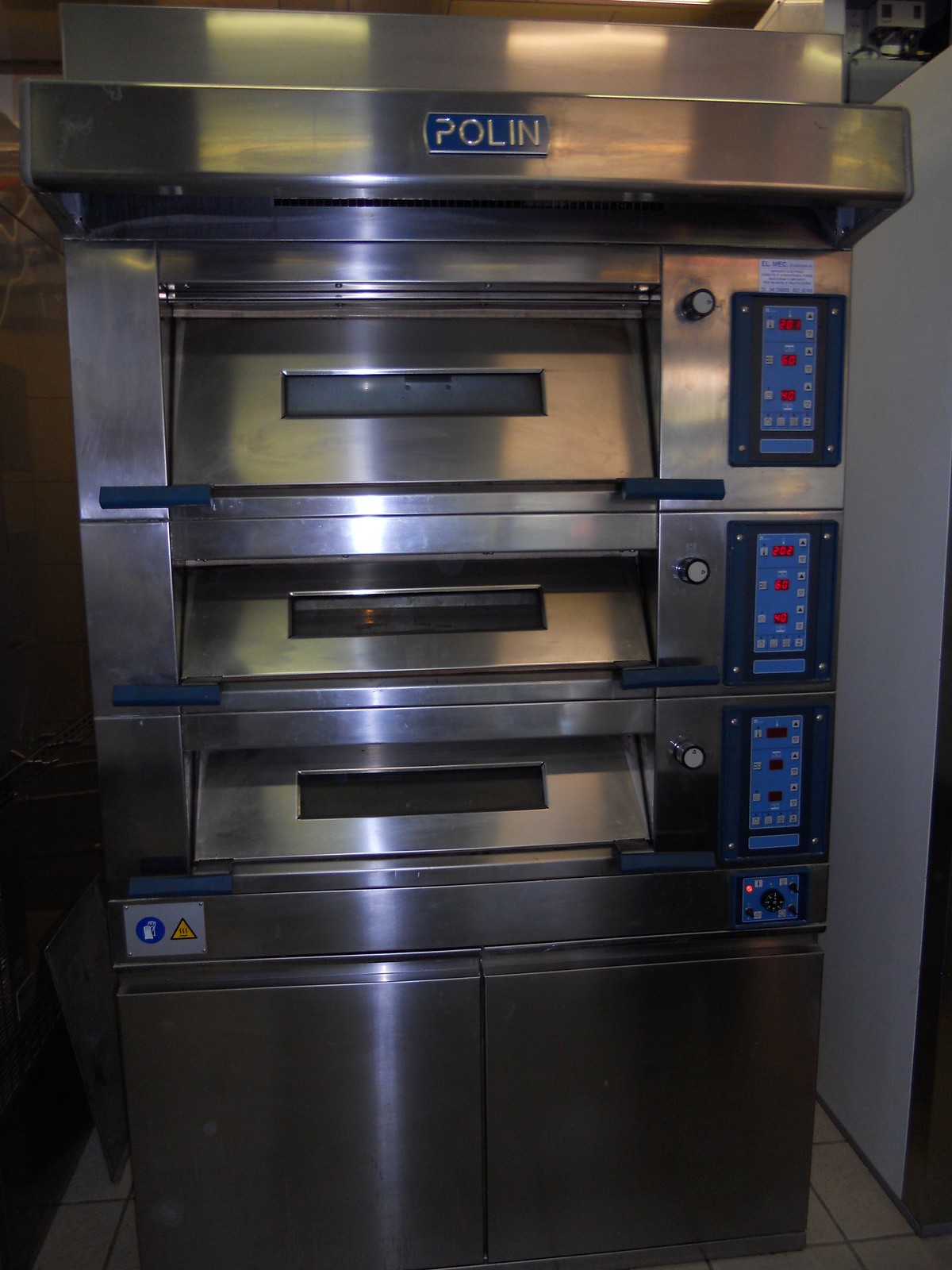The image depicts a high-end industrial oven by Polin, characterized by its stainless steel construction. This sizable appliance features three stacked oven compartments, each with a black pull handle and a small rectangular viewing window. The top compartment is slightly taller than the bottom two. Flanked by a blue control panel with red indicator lights and round knobs, the oven’s settings are managed from this interface. Below the trio of ovens, the unit incorporates two stainless steel French-style (double) doors, likely intended for storage. A conspicuous yellow hazard symbol is noted near the bottom controls. The device is positioned on a yellow-tiled floor against a white wall with a brown trim, suggesting its placement in a commercial kitchen environment. The branding 'Polin,' in blue lettering, is mounted prominently on a tag at the top of the unit.